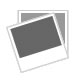This is a top-down photograph of an old, vintage container, reminiscent of a kitchen sugar pot. The container features a predominantly silver, metallic lid characterized by age marks, scratches, and slight rust, giving it an antique charm. Central to the lid is a round nub for lifting it, flanked by intricately designed handles made of two intertwining, zigzagging pieces of metal that form oval loops. The body of the pot, though partly obscured in the photo, is a faded pink adorned with images of red flowers and subtle black patterns. The container rests on a white cotton tablecloth, further enhancing its nostalgic, vintage appeal.